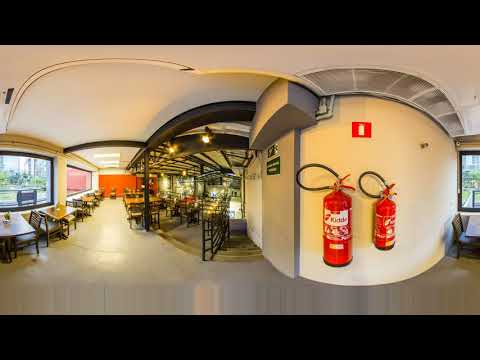This panoramic photograph captures the interior of an eating establishment, possibly a cafeteria or restaurant. The ceiling is painted white and features a mix of directional light fixtures and square, recessed LED lights that illuminate the space. The room is furnished with multiple square and rectangular tables, each with seats on both sides and what appear to be napkins and condiments in the center. The left wall is dominated by large windows that let in natural light, indicative of daytime, while the right wall is noted for its two prominent red fire extinguishers, one identified as a product from the company KIDDE, alongside a smaller window partly obscured by poles. The central area of the image reveals stairs descending to a lower level, and metal railings lead towards a serving area where food can be obtained. Despite the slight distortion from the panoramic capture, the overall layout appears to be a long, spacious room, with off-white floors and walls that carry a yellowish hue.